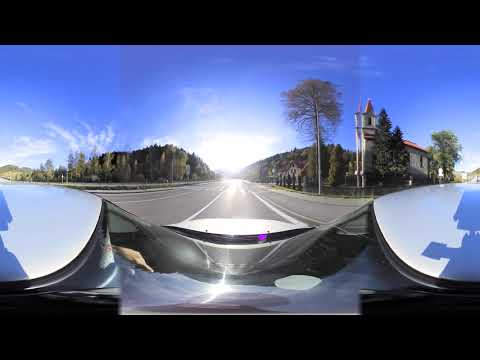The image showcases a highly distorted fisheye view from a 360 camera mounted on top of a vehicle, possibly a car. The warped perspective prominently features both the front windshield and roof of the car, with visible details such as the hand of the driver on the left-hand side. The road ahead is a gray, multi-lane blacktop with white lines, set under a bright, blue sky with wispy white clouds. The sun is shining directly, illuminating the entire scene.

On both sides of the road, there are dense sections of tall, green trees, complemented by some rolling hills on the left. The right side of the image reveals a striking large tree that stands out among the others, along with a building that has a distinctive cone-shaped tower and white siding. This building also features red clay-colored roofs and is surrounded by a fence. Horizontal black strips run across the top and bottom edges of the image, adding to the visual distortion and emphasizing the surreal, twisted nature of the fisheye perspective.